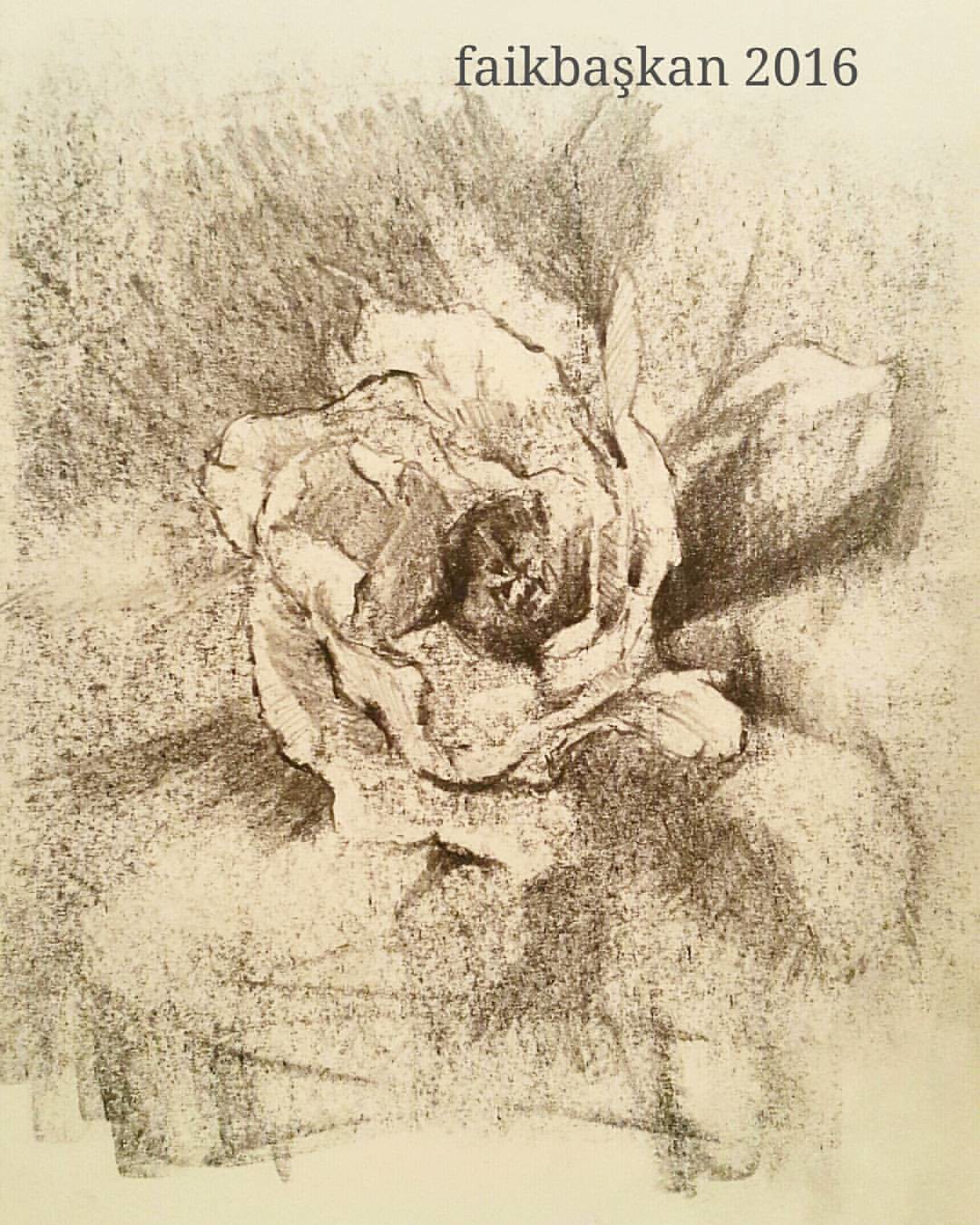In this detailed black and white drawing, an intricately sketched rose takes center stage on an off-white piece of paper. The core of the rose is rendered in a deep black, sharply contrasting with the white petals delicately shaded with touches of gray. Surrounding the flower, there is additional black shading, suggestive of pencil work, which adds depth and texture to the composition. 

In the top right corner of the drawing, the word "FAIKBASKAN" is inscribed in capital letters alongside the year "2016," possibly indicating the artist's name and the year of creation. Subtle horizontal lines are present beneath the rose, contributing to the background detail and balance of the artwork. On the right side, two larger white petals edged with black shadows appear, potentially acting as a visual echo or shadow of the primary flower, enhancing the complexity and dimension of the drawing.